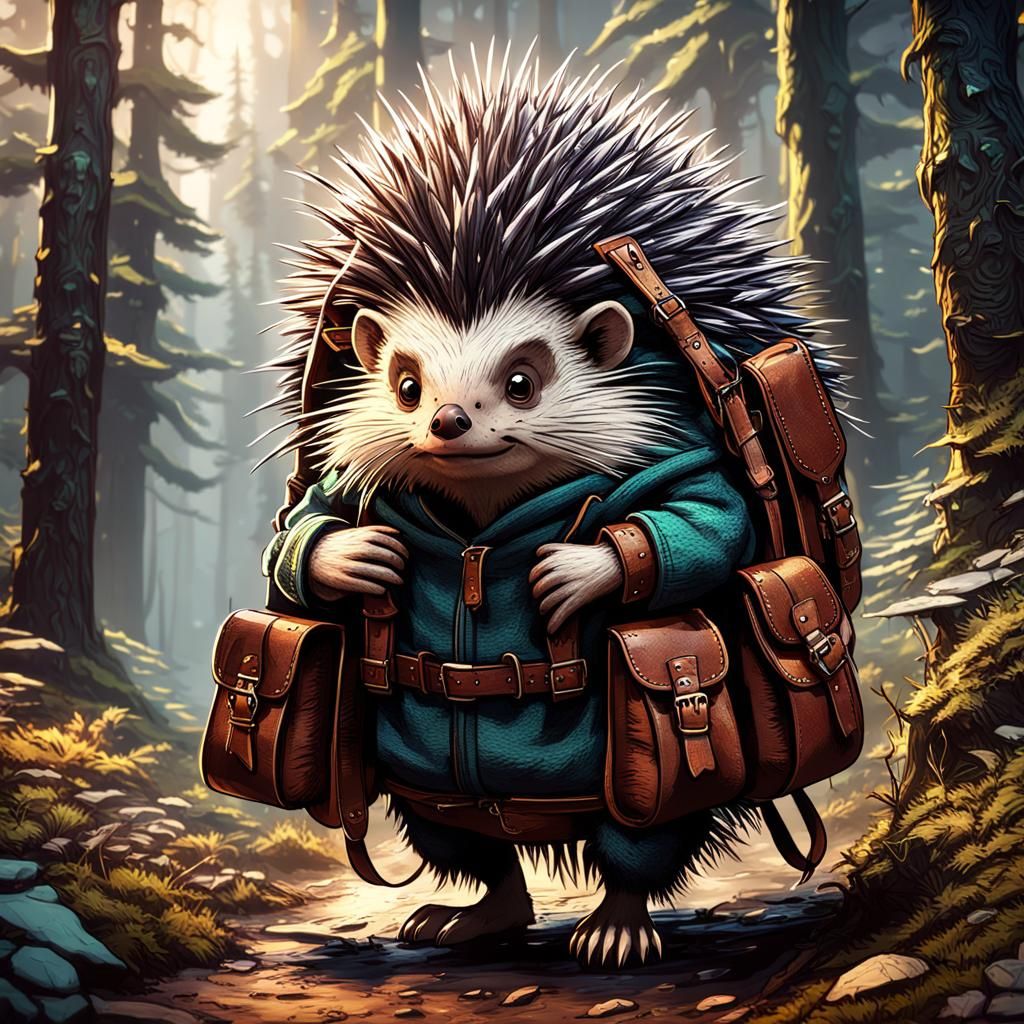The detailed illustration presents a whimsical scene that feels reminiscent of a children's storybook. It features a large porcupine walking upright on a dirt path through a dense forest of tall, brown trees. The porcupine is dressed in a teal green hoodie, with the hood down, revealing its spiky quills. Adorned in a brown leather belt, it carries multiple gray leather pouches and a large matching brown backpack, suggesting a creature on a journey. The path beneath its feet is a mix of dirt, stones, and gravel, with occasional pebbles and small plants. Small mushrooms and other foliage dot the sides of the trail, and patches of sunlight filter through the trees, adding a magical touch to the serene woodland setting. The porcupine's legs are covered in dark fur, complementing its overall earthy and natural color palette.